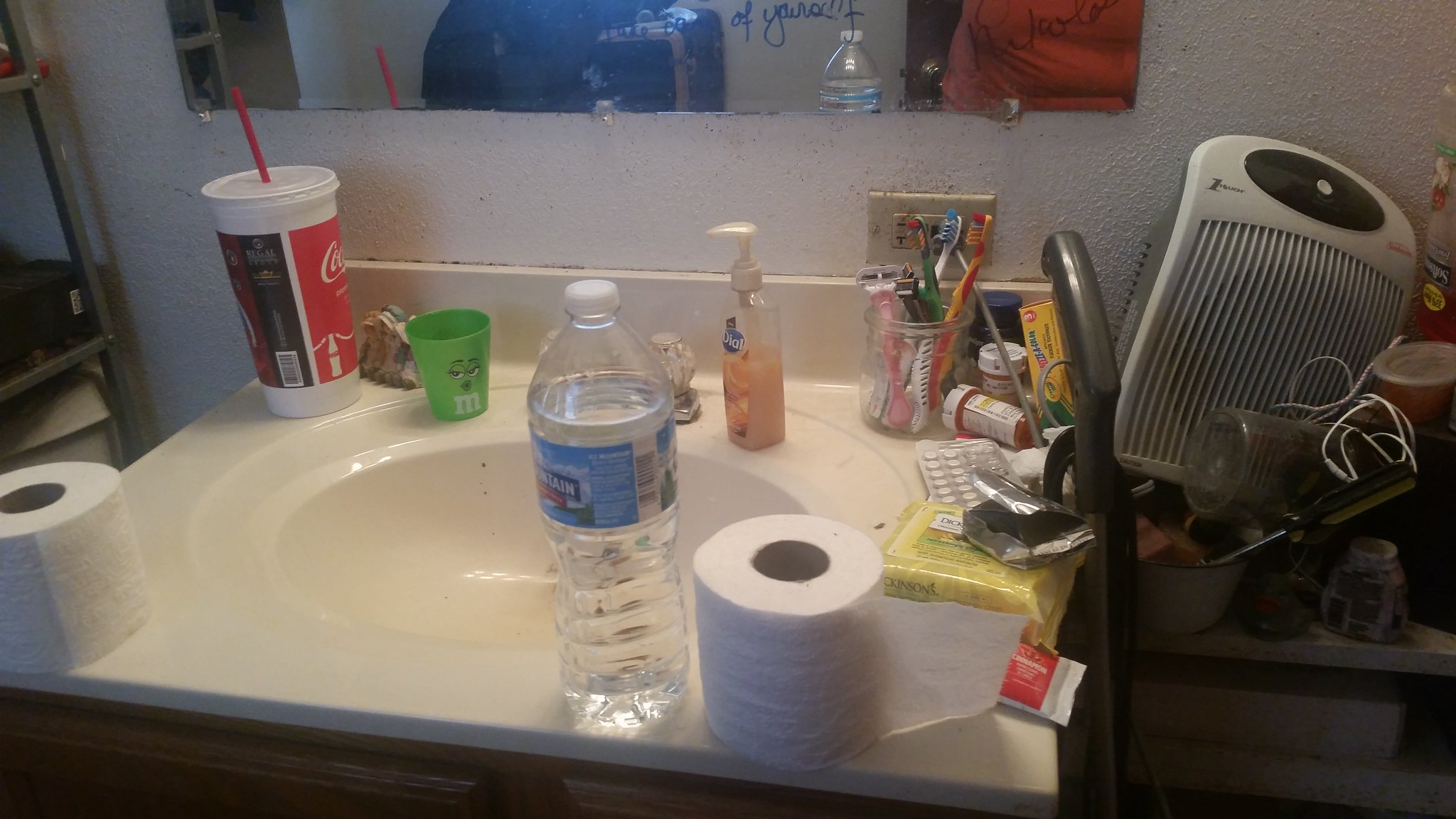On a cluttered bathroom countertop, the scene is set as follows: 

Against a popcorn-white wall backdrop, a notably messy sink area is captured. At the forefront, a roll of toilet paper sits at the bottom left corner of the countertop. Just to the left, there's a blue M&M's cup along with a Coca-Cola soft drink placed on the counter. Dominating the central area is a water bottle, partially obscuring the faucet of the sink. 

To the right, a peach-scented hand soap dispenser is placed near the edge. Adjacent to it, a collection of pills is scattered on the surface. Further right, resting against the wall, is a white fan or heater, currently not in use. An organized clutter of various items, including a cup holding toothbrushes, populates the metal shelf hanging on the back wall. 

Above, a mirror reflects the scene, adding depth to the already crowded space. In the middle right area, the handle of what seems to be a vacuum cleaner or another long object juts out. The overall impression conveyed is one of a heavily used and somewhat chaotic indoor bathroom sink area.